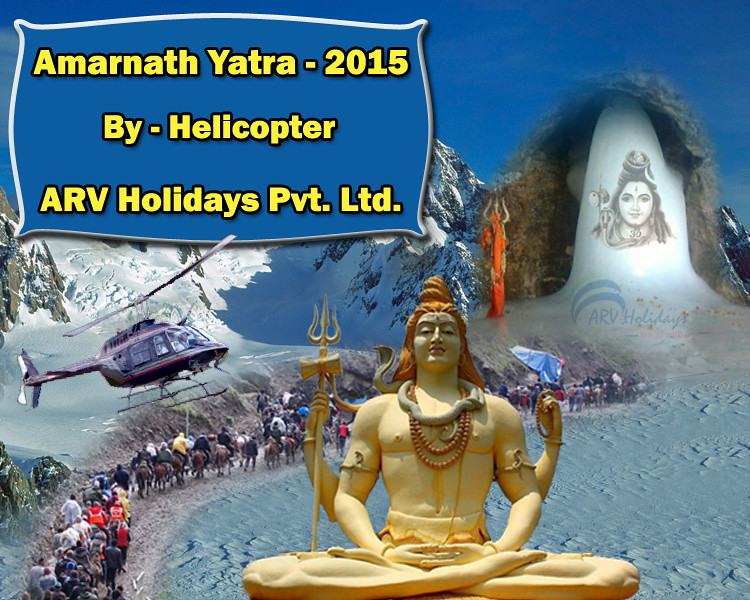The image is a vibrant, detailed color collage in landscape orientation, designed as an advertisement poster. It prominently features depictions from a pilgrimage event known as Amarnath Yatra 2015 by Helicopter, promoted by ARV Holidays Pvt. Ltd., as stated in a twisted white rectangle with yellow text on the upper left.

The foreground showcases a large, seated statue of Lord Shiva, a central figure in Hinduism, adorned with long red hair and beaded necklaces. Shiva sits cross-legged, hands positioned at his sides holding a Trishul (trident) and prayer beads. There are snakes coiled around his upper arms and neck, enhancing the divine imagery.

On the lower part of the poster, in the middle, devotees are shown traversing a snow-laden mountainous path. Some are on foot, while others ride on mules or horses, all making a pilgrimage towards a sacred ice formation resembling a Shiva Linga, which symbolizes Shiva in Hindu tradition. 

In the background, towering snowy peaks, likely representing the Himalayas, add to the dramatic and spiritual setting. Mounted on top of these peaks is a cutout image of a helicopter, signifying the mode of transportation for the pilgrimage.

On the right side of the image, there is a black-and-white sketch of Shiva's face, echoing the deity's prominence found in the middle of the collage. Overall, the image employs a photographic realism style, using special filters and techniques to blend different elements into a cohesive and picturesque portrayal of the Amarnath Yatra pilgrimage.